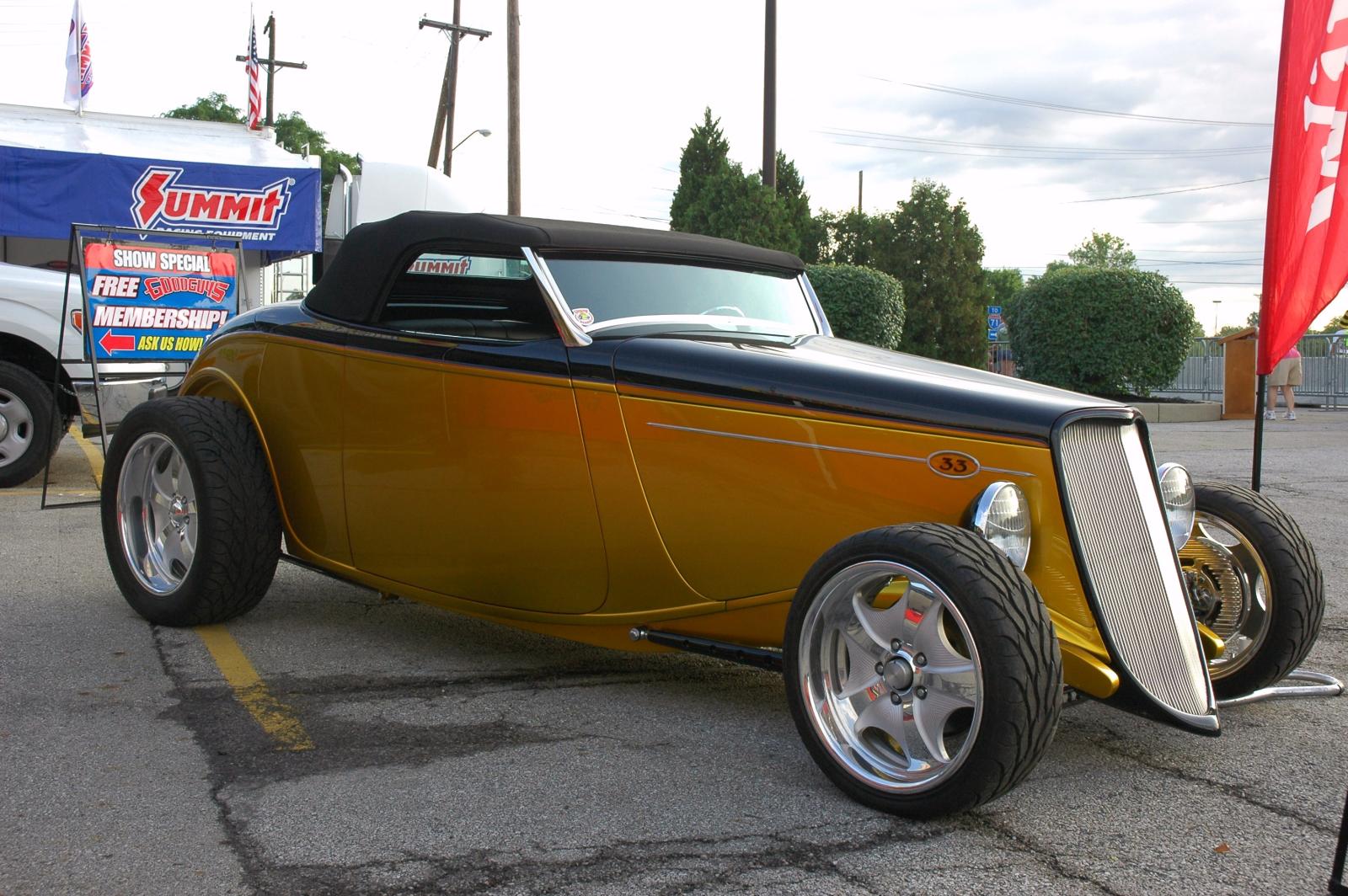An old vintage car, predominantly yellow with hints of greenish-yellow and possibly a chameleon-like effect reflecting shades of gold and orange, is parked on an asphalt lot. This narrow car features an elongated, skinny hood and widens towards the back, sporting a two-seater layout. It has a distinctive black fabric convertible top that stretches from the hood to the rear. The front end of the vehicle is white, accentuating its unique color palette, and it stands on small wheels that seem mismatched and outside the typical size for such a classic car. In the parking lot around the car, there is a notable red flag with white text that mentions a "Summit free membership." The background reveals a mix of visual elements: a white sky with grey clouds, trees, bushes, power lines, crosses, and American flags. Additionally, a blue sign on a white tan structure is visible behind the car.